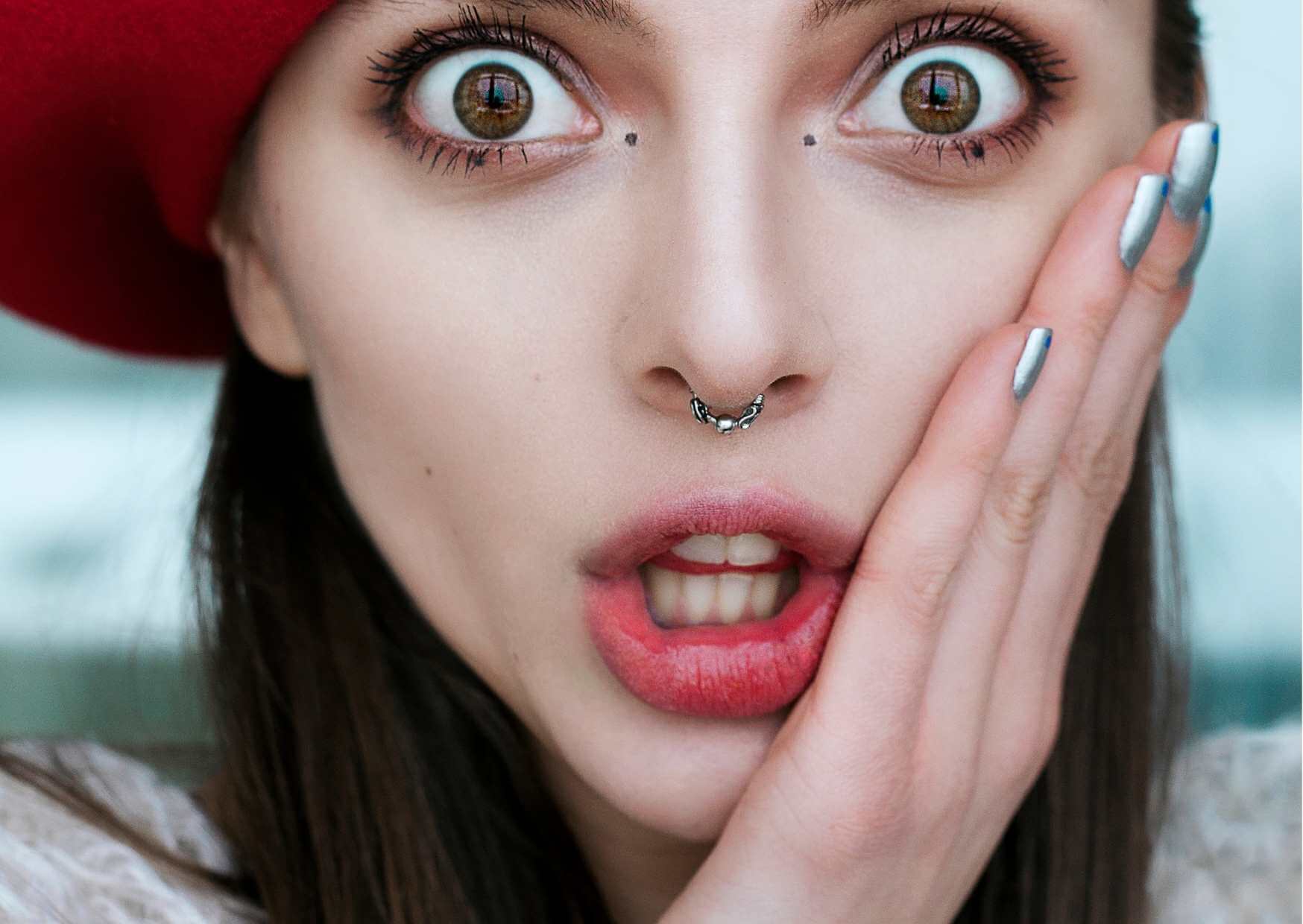The close-up image features a pale-skinned woman with a thin, gaunt face, striking a dramatic and obviously fake shocked expression. Her wide, brown-hazel eyes are accentuated with eyeshadow, mascara, and painted black dots near the corners and below them. Her lips, adorned with pinkish-red lip gloss, are perched slightly open, revealing her teeth. She has dark brown hair, partially covered by a red beret, and wears a gray sweater. Her left hand, decorated with metallic gray nails tipped with blue dots, rests against her cheek, enhancing the expression of surprise. The woman also sports a silver septum ring connecting her nostrils. Blurred in the background are hues of blue, gray, and green, directing full attention to her theatrically shocked visage, suggestive of a staged or stock photo. The overall impression hints at an advertisement or artistically posed image.